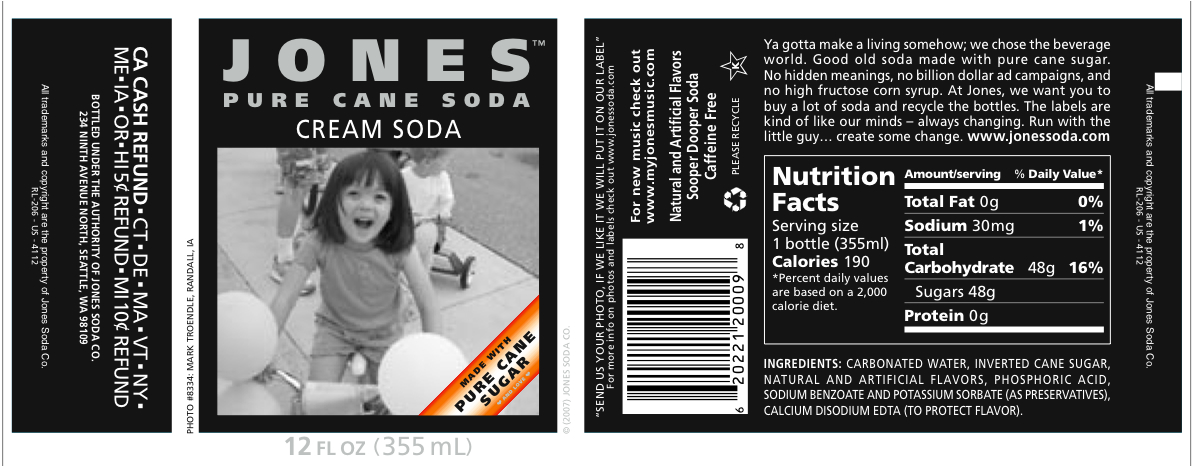This image showcases a flat, unwrapped label of Jones Pure Cane Soda Cream Soda. The overall background of the label is black with light-colored gray and white lettering. The front section prominently displays "Jones Pure Cane Soda Cream Soda" in gray letters, accompanied by a black-and-white photograph of a smiling little girl on a tricycle. Behind the girl, two other children on tricycles are slightly visible, enhancing the playful scene. Diagonally across the picture, from bottom center to top right, an orange banner states "Made with Pure Cane Sugar" in black letters. To the left, in a vertical format, white lettering on the black background provides refund information by listing states alongside their specific refund amounts. On the right side, the remaining part of the label includes the Nutrition Facts panel and a list of ingredients in white lettering. Additionally, the label contains a barcode and information indicating it is bottled under the authority of Jones Soda Company.